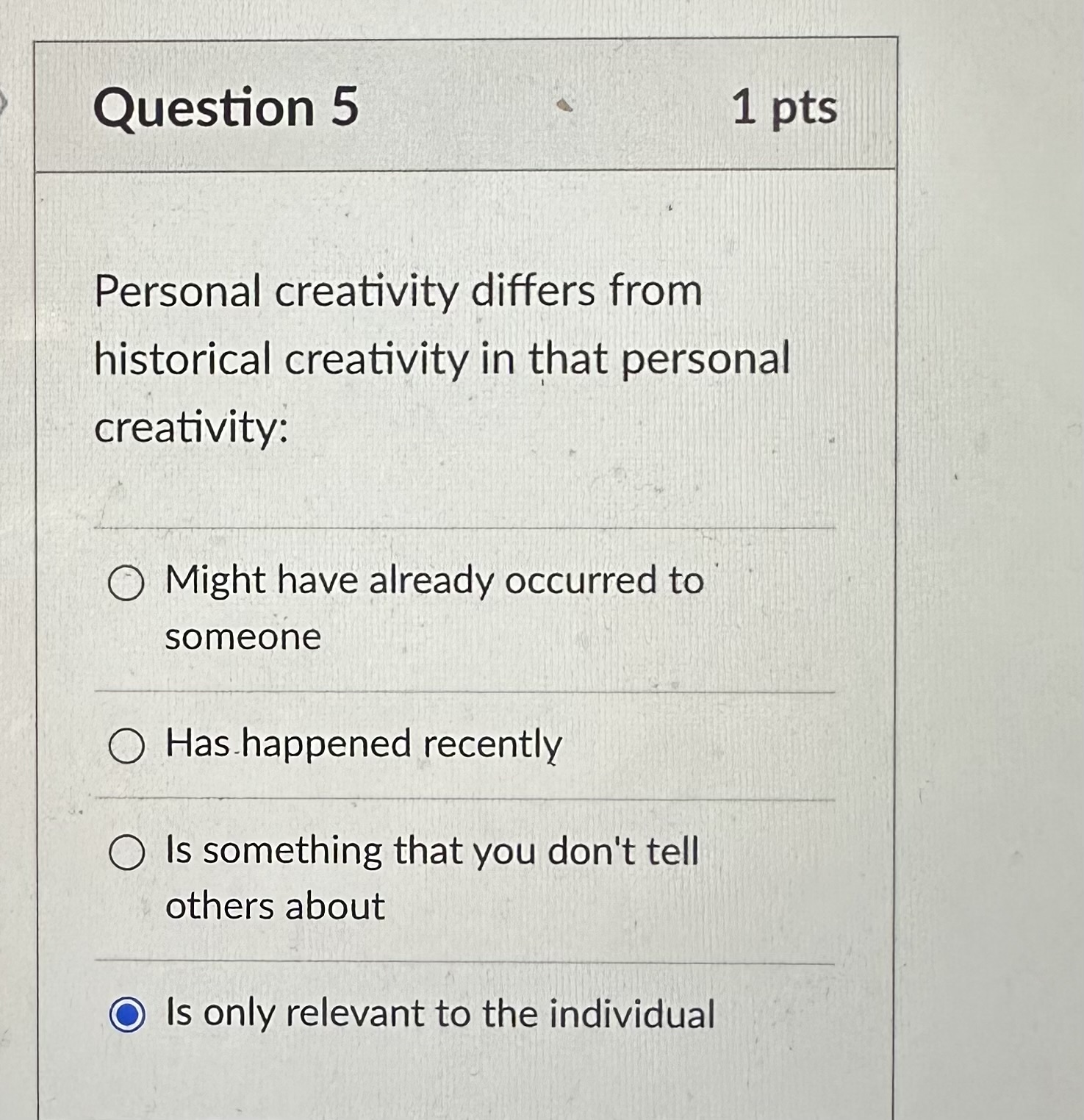The image displays a screenshot of a quiz interface, likely from a test site. The background is a uniform shade of gray, providing a neutral canvas for the quiz content. At the top of the screenshot, in bold black text, is the heading "Question 5 worth one point." The question posed reads, "Personal creativity differs from historical creativity in that personal creativity," followed by four multiple-choice options. 

The selected option, highlighted in blue with a corresponding circular indicator, states "is only relevant to the individual." The three unselected options are:
- "might have already occurred to somebody,"
- "has already happened recently," 
- "is something that you don't tell others about."

All text is rendered in a clear black font, ensuring readability against the gray background. The only other color present on the page is the blue used for highlighting the selected answer, which stands out distinctly against the monochrome scheme. The perspective of the screenshot suggests it was captured from a screen, either a computer or a mobile device.